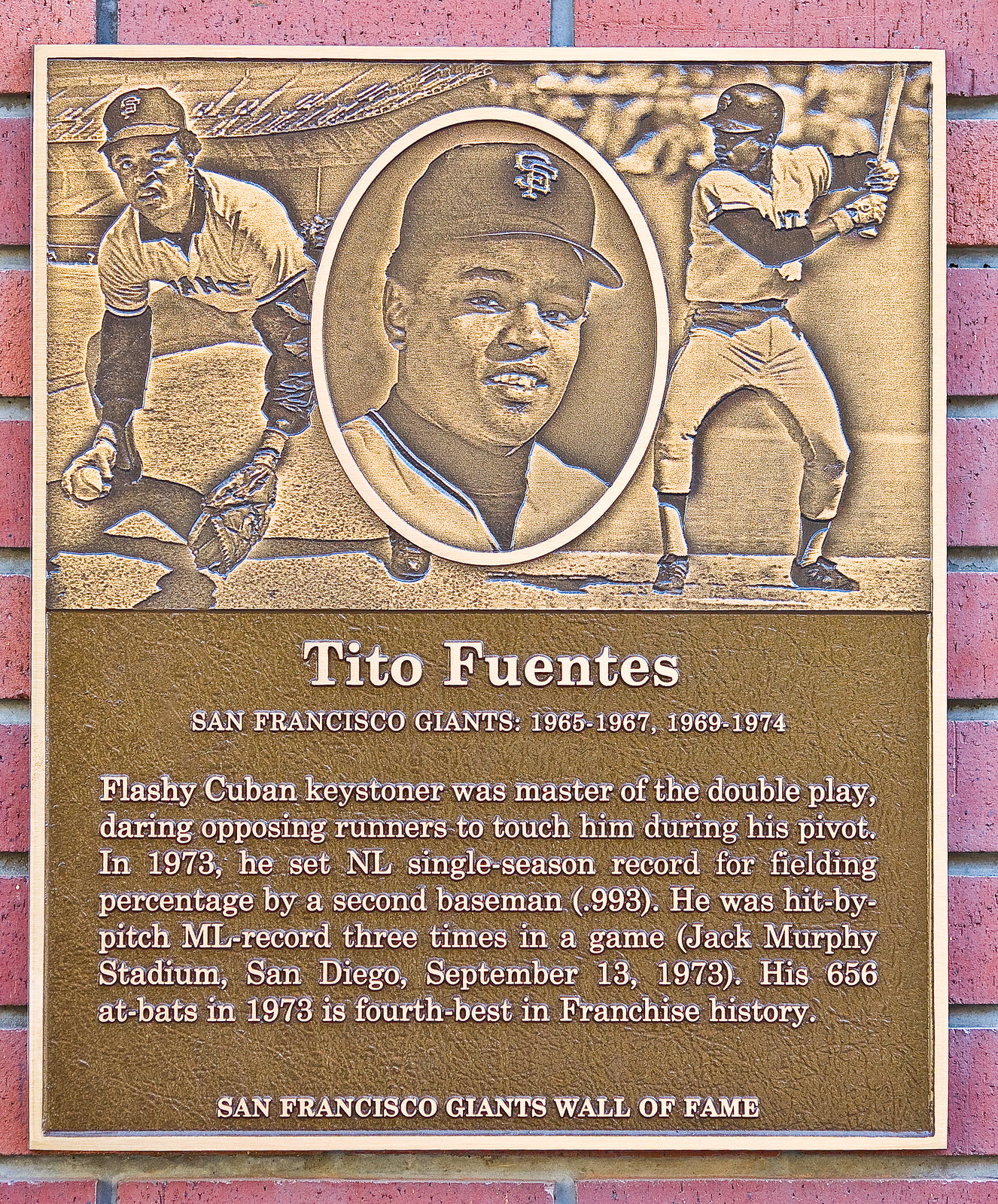This image captures a bronze plaque mounted on a reddish brick wall, commemorating Tito Fuentes, a notable second baseman for the San Francisco Giants. The plaque features three distinct images at the top: on the left, Fuentes is depicted in a defensive stance, likely fielding a ground ball; the center image is an oval close-up of his face, reminiscent of a baseball card; and on the right, he is shown in his distinctive batting stance. Below the images, the text celebrates Fuentes’ career with the Giants, highlighting his tenure from 1965-67 and 1969-74. It describes him as a "Flashy Cuban Keystoner" and a master of the double play, noting his daring pivots. Notably, in 1973, Fuentes set the National League single-season record for fielding percentage by a second baseman at .993 and was hit by pitch a major league record three times in one game at Jack Murphy Stadium, San Diego, on September 13, 1973. His 656 at-bats that season rank among the best in the franchise's history. The plaque concludes by noting it is part of the "San Francisco Giants Wall of Fame."